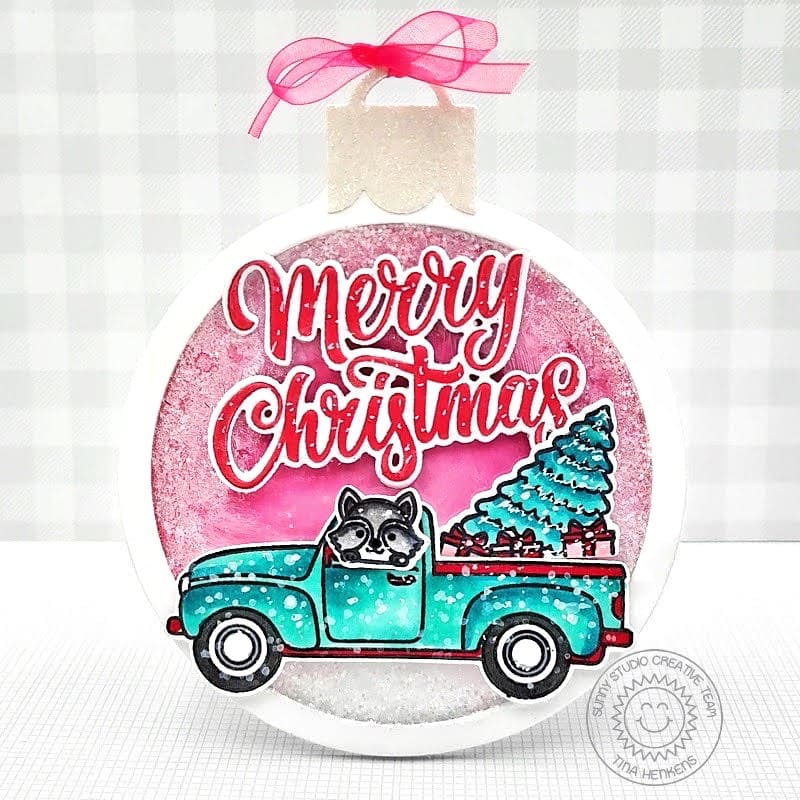The image showcases a festive, round item resembling a Christmas ornament or possibly a bag with a handle that mimics a padlock. At the top of the ornament, a pink ribbon is tied around the handle. The ornament itself is silver with a red insert and features the cheerful phrase "Merry Christmas" in red cursive text with a white border. Displayed prominently is a green truck, carrying a Christmas tree and multiple presents in its bed, with a raccoon sticking its head out from the driver's side. The edges of the item are bordered in white, giving it a snow globe-like appearance. In the bottom-right corner, the words "Sony Studio Creative Team, Tina Hickens" are inscribed. The background of the image is a white gingham pattern, adding to the holiday charm.